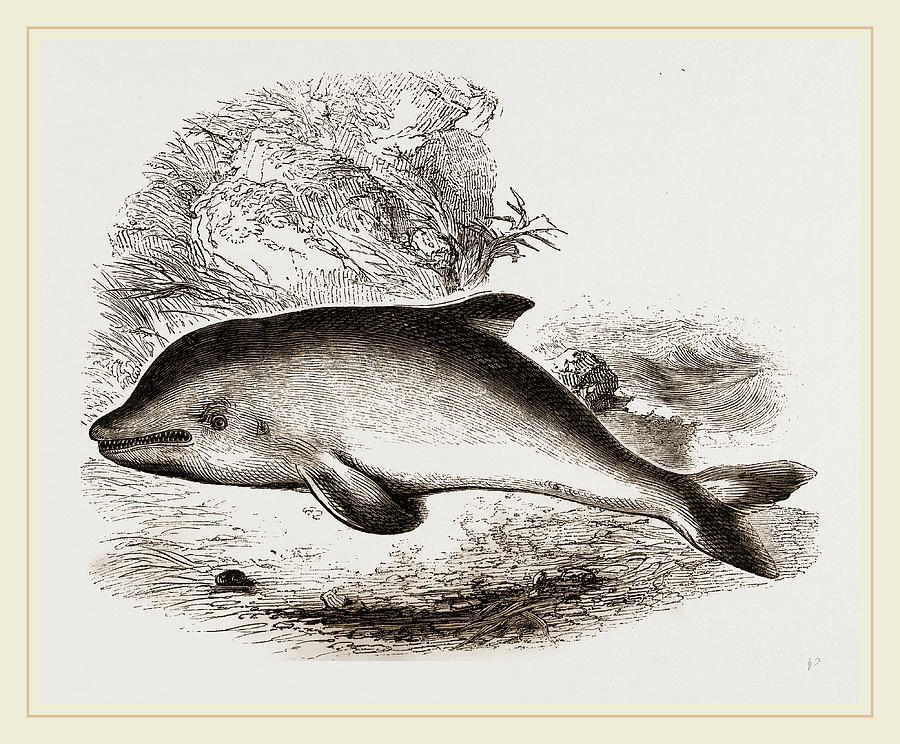This is an intricately detailed black and white pencil or pen drawing of a dolphin-like aquatic mammal, possibly from a prehistoric era or an artist's imaginative rendition, characterized by a more robust body than a typical dolphin. The creature is depicted on its side, showcasing its rounded body with shading details that highlight a darker top and a lighter underside. It possesses a top fin, one visible side flipper, both tail fins, beady eyes with a slight raised eyebrow expression, and a pronounced grin baring its teeth, evoking a growling dog's snarl.

The drawing's backdrop features a roughly sketched rocky cliff adorned with craggy grasses and plant life, suggesting a coastal or shallow underwater environment. The meticulous shading and scratch marks around the dolphin imply a shadow beneath it, emphasizing its position in shallow waters where light penetrates. The entire composition is rendered on white paper bordered by a light beige frame, completed with a distinct red line dividing the white paper from the beige border, adding a touch of color to the overall monochrome artwork.